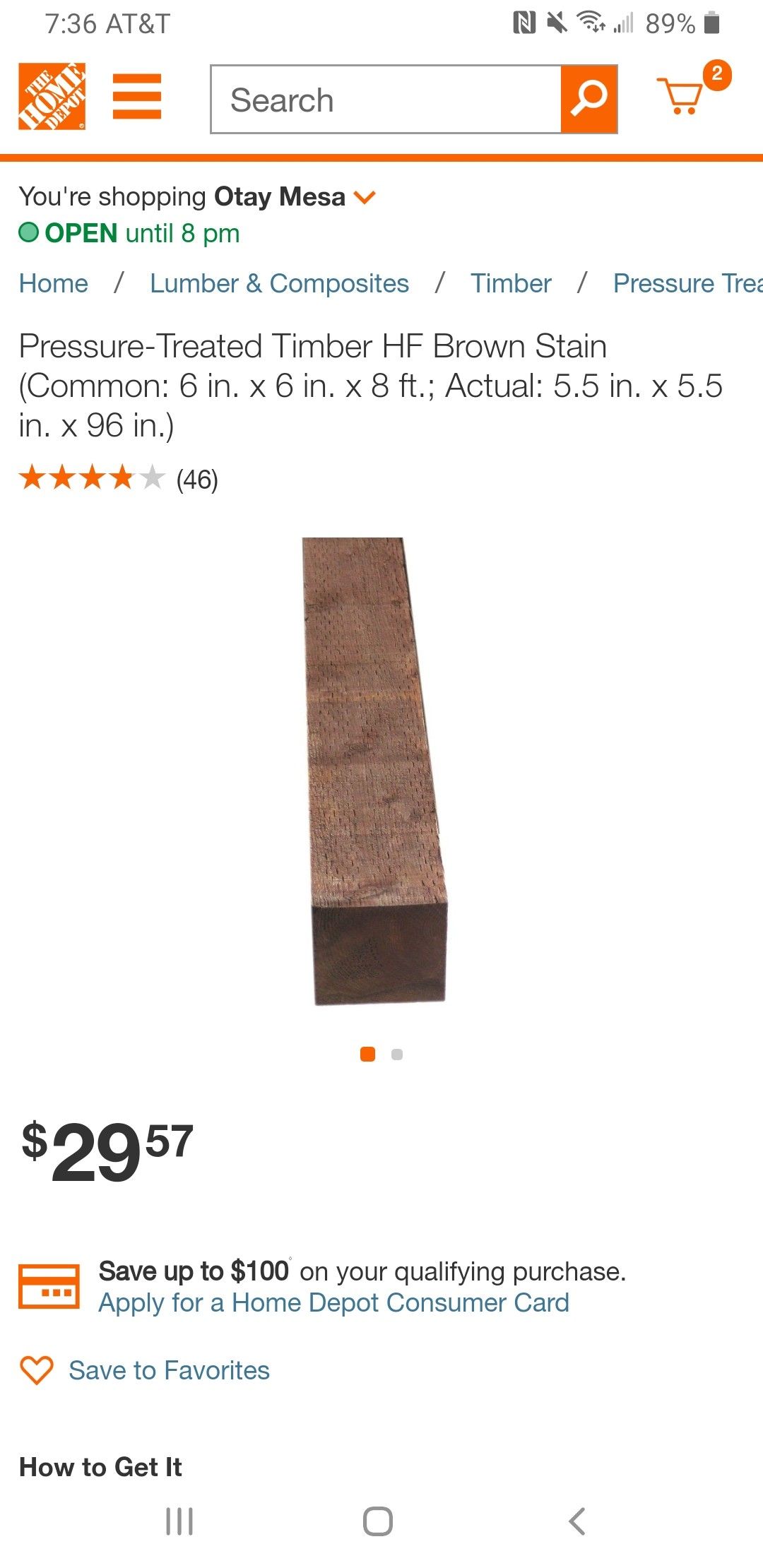This is a detailed screenshot of the Home Depot website on a mobile device. In the top left corner, the distinctive Home Depot logo is displayed, featuring the store's name in white text set at an angle within an orange square. To the right of the logo, there's an orange menu button symbolized by three horizontal bars. Next, there's a prominent search bar accompanied by an orange search button. Further to the right, an orange shopping cart icon indicates that there are two items added to the cart. 

Directly below this header section, a thin orange line separates the navigation bar from the rest of the content. Beneath, in bold text, it states, "You're shopping Mesa," accompanied by a drop-down menu. There is also a status message in green text stating, "Open until 8 p.m."

Just below this, a navigation menu contains four links: "Home," "Lumber," and "Composites," followed by "Timber," and finally, "Pressured," though this last word is cut off.